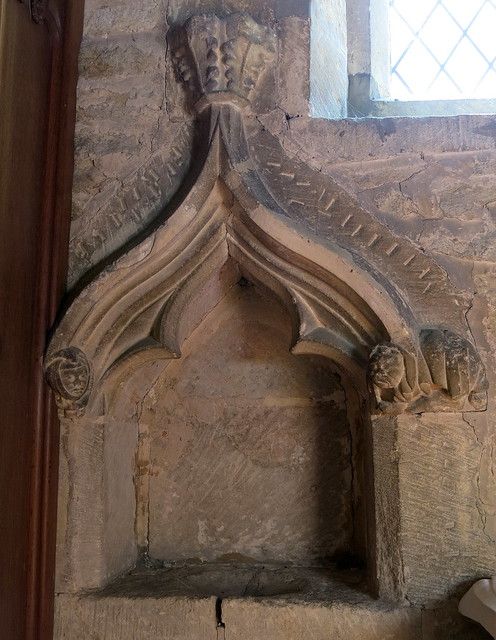This photograph captures an aged, ornate interior scene, likely within a historic church or cathedral, emphasized by the stone walls that evoke a sense of antiquity. Central to the image is an intricately designed, arched niche set into the stone wall, featuring a bowl-shaped basin at its base, possibly intended to hold holy water. The arch of the niche is adorned with detailed carvings, including faces and perhaps animal motifs, culminating in a crown-like ornamentation at the top. The overall coloration of the stone wall has a weathered, stucco-like appearance. Partially visible on the left side of the photo is a section made entirely of wood, contrasting with the surrounding stone. The top right corner reveals a small window with diamond-pane glass and metal criss-cross bars, adding to the historic atmosphere of the scene.